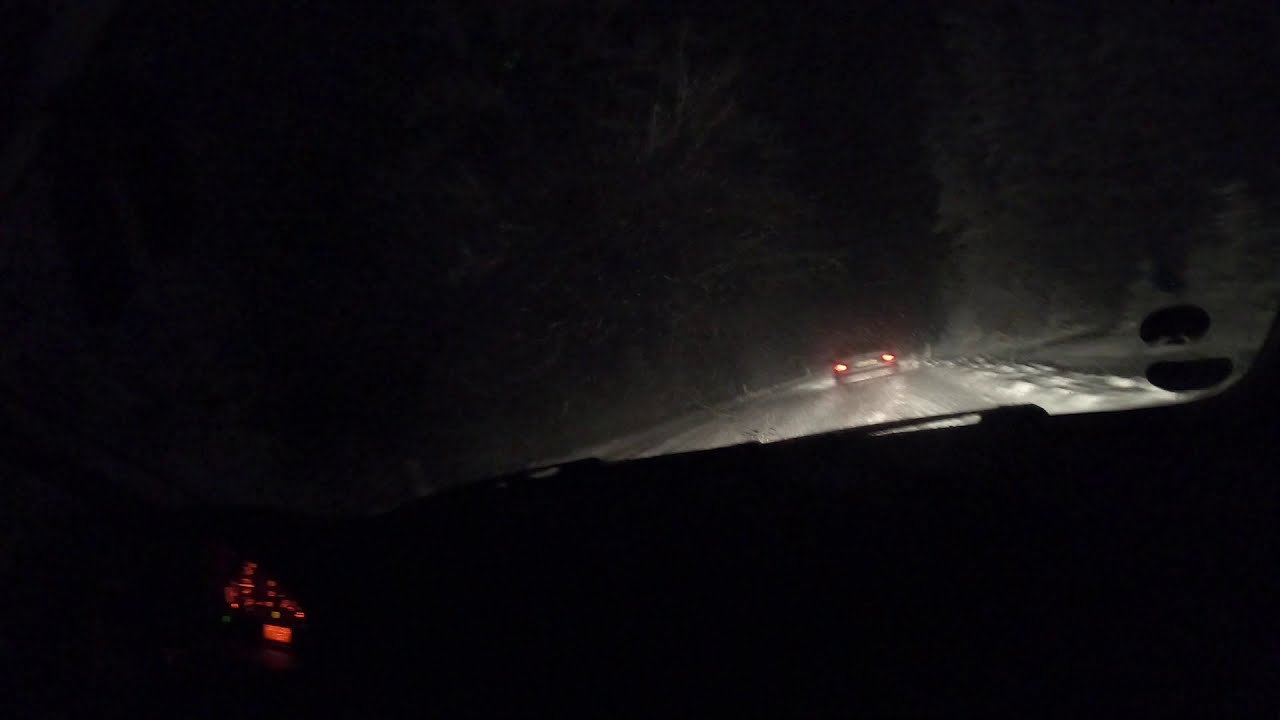The photo captures a nighttime scene taken from inside a car through its windshield. The image is dark and somewhat blurry, with the bottom half mostly solid black, likely due to the windshield wipers resting at the base of the windshield. The glowing digital odometer and a hint of the steering wheel are visible on the lower left side. The car's headlights illuminate the road ahead, revealing snow-covered ground and dense evergreen trees lining both sides. Directly in front, the red taillights of another car, a grayish sedan, cast an eerie glow, adding to the spooky ambiance. The snowy road and the silhouetted trees enhance the sense of isolation and darkness. Small stickers can be seen on the bottom right of the windshield, completing the scene from this dimly lit interior.